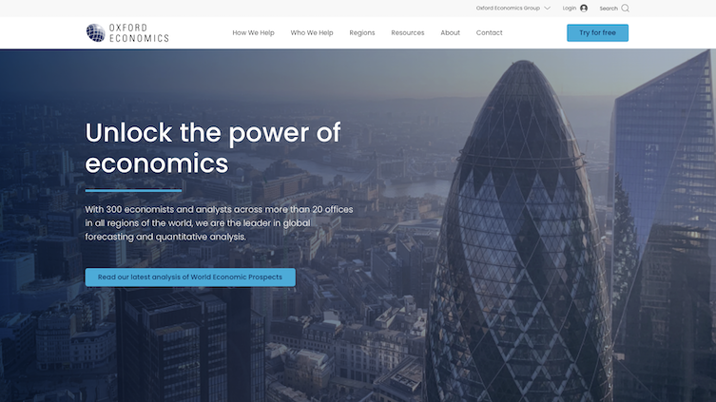Screenshot of the Oxford Economics website:

The screenshot captures the Oxford Economics website. At the top left, the logo features a stylized sphere with a grid overlay and a specular highlight. The words "Oxford" and "Economics" are stacked vertically in simple, condensed text with wide kerning on a white bar. The navigation menu includes the following options: "How We Help," "Who We Help," "Regions," "Resources," "About," and "Contact." A light blue "Try for Free" button is positioned at the top right, alongside options for "Login," "Search," and "Oxford Economic Groups" with a dropdown menu.

Dominating the page is a large hero image of the iconic glass structure resembling a Fabergé egg, known as the Gherkin in London. The aerial shot, taken on a hazy day, shows the London Bridge and Tower Bridge faintly in the background. A subtle haze overlay darkens the image, enhancing the readability of the text.

In white text, the main headline reads, "Unlock the power of economics," followed by a thin blue line. Beneath it, a subheadline states, "With 300 economists and analysts across more than 20 offices in all regions of the world, we are the leader in global forecasting and quantitative analysis." A prominent wide blue call-to-action button encourages visitors to "Read our latest analysis of world economic prospects."